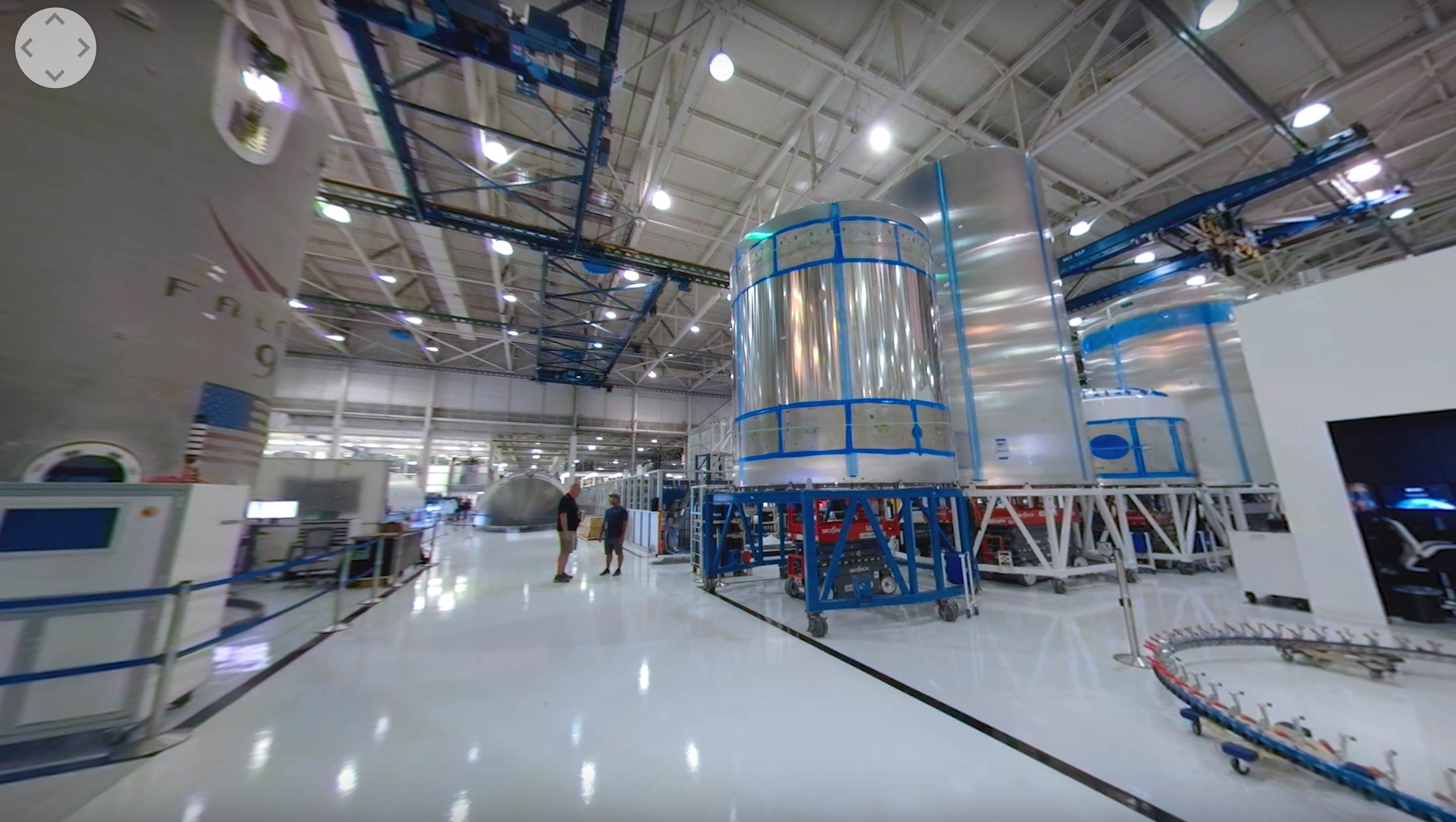The image depicts the interior of a spacious, well-lit warehouse or manufacturing facility, likely part of SpaceX's operations given the prominent "Falcon 9" cylinder towards the right. In the center of the image, two men are conversing; the first man wears a black t-shirt, brown shorts, and shoes, while the second man, sporting a cap, blue shirt, shorts, shoes, and a name tag, stands beside him. Their surroundings feature a shiny, white floor reflecting the ceiling lights, and an array of blue and white railings overhead. A large cylindrical tube dominates the central part of the image, and to its right, a bordered-off section contains another cylinder placed on a hydraulic, movable metal shelf. An American flag is subtly visible, further emphasizing the high-tech, pristine environment of the facility.